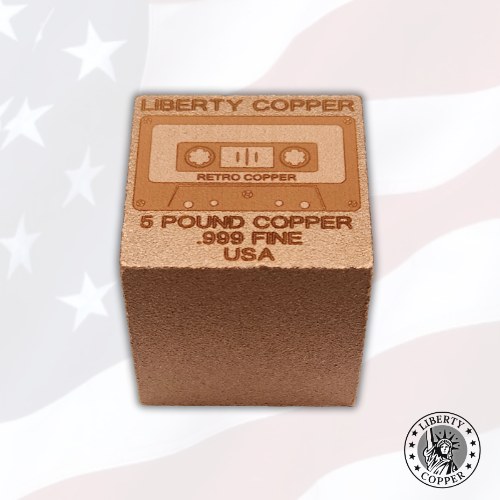This image features a prominent copper-colored cube that serves as the focal point. The top surface of the cube prominently displays the words "Liberty Copper." Below this, an engraved design reminiscent of an old videocassette tape is labeled "Retro Copper," complete with two circles where the tape reels would be. Further details on the cube include the text "5 pound copper, 0.999 fine" and "USA." The backdrop is a very pale and faded rendition of the American flag, with indistinct stripes and stars. In the bottom-right corner of the image, there is a small circular emblem. The emblem is bordered with the words "Liberty" at the top and "Copper" at the bottom, and it features an image of the Statue of Liberty in the center.